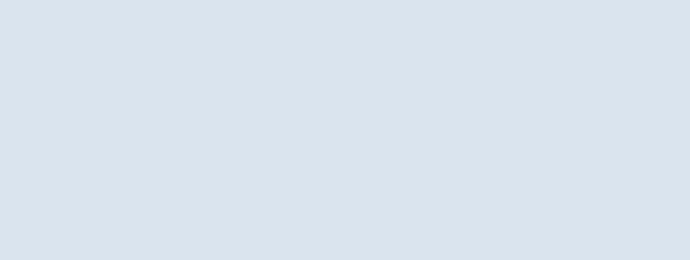This image showcases a rectangular box with its longer side oriented horizontally from left to right. The box is colored in a subtle bluish-gray hue, devoid of any additional features or contents. The horizontal length of the rectangle appears to be at least twice as long as its vertical height, emphasizing its elongated shape.